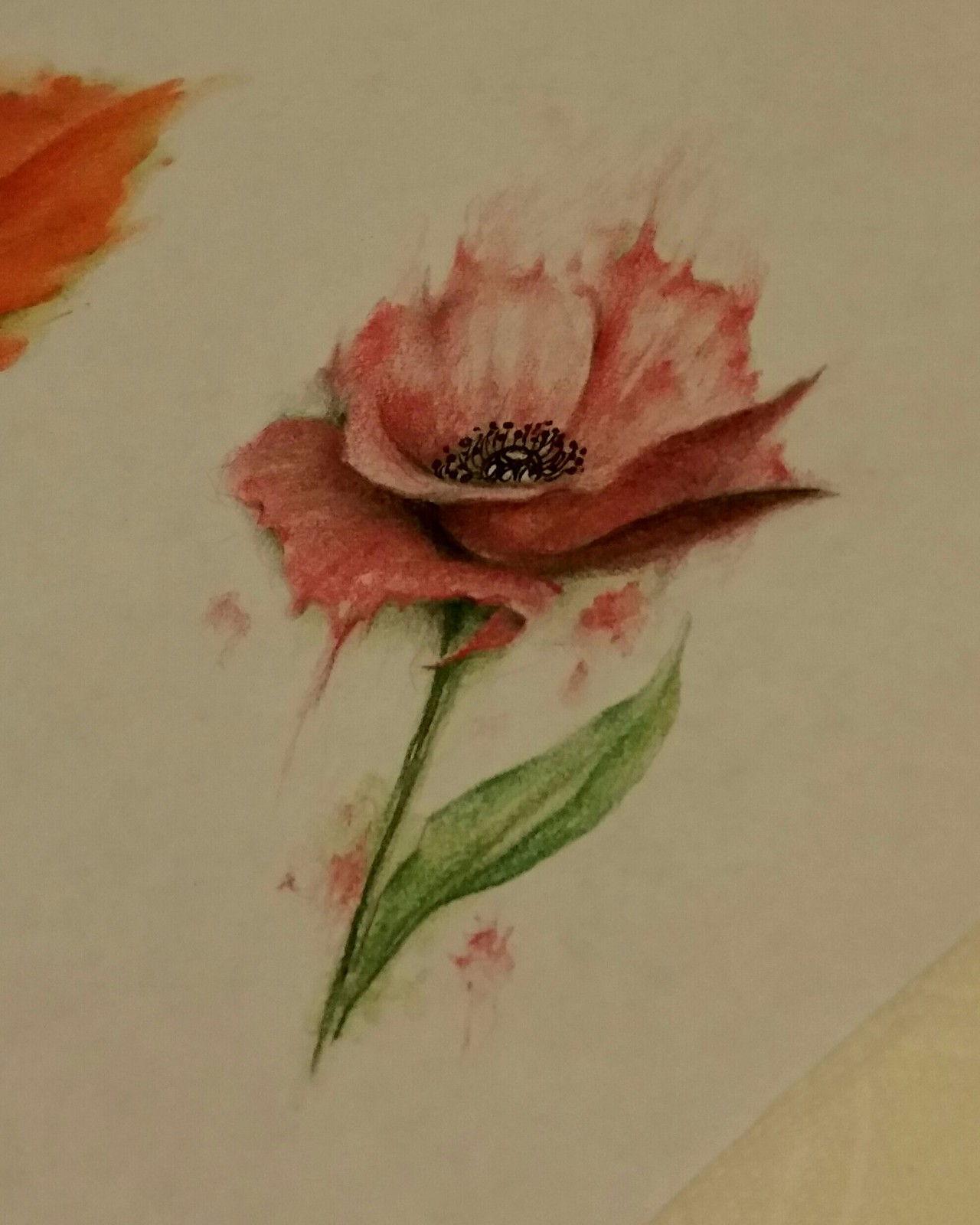An exquisite watercolor painting depicts a single flower against a subtly pale gray background, suggesting the texture of delicate paper. This ethereal blossom features a slender, verdant green stem and a long, thin leaf of a matching hue. The flower itself radiates in a serene pinkish-gray tone, its petals arranged in layers: an outer ring of two to three petals gives way to an inner cluster of lighter pink and white blooms. At the heart of this floral marvel, the intricate details of the stigma and stamen are meticulously rendered. Enhancing the composition, gentle pink smudges cascade down below the flower and extend from the petals, adding an enchanting, almost whimsical touch to the overall beauty of the painting.